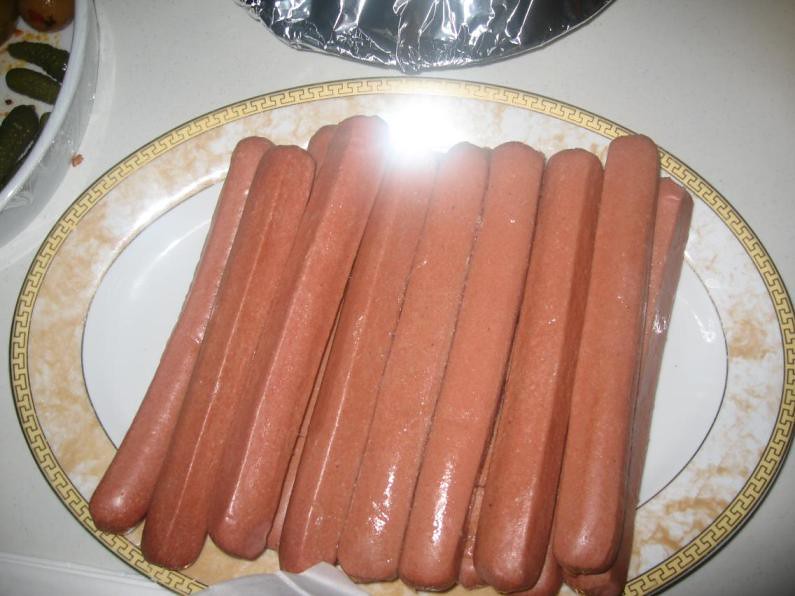This detailed indoor image focuses on a close-up view of a white marble-like ceramic platter with an opal shape, adorned by a thin gold and brown embroidered border. Stacked vertically and piled three layers deep in the center of the platter are about 15 pink hot dogs. The platter appears to have a small chip along its bottom edge. The hot dogs cover most of the plate's length, with light from above reflecting off their tops and a nearby aluminum foil-covered dish. The photograph is taken from a top-down perspective, showcasing the platter on a white countertop. To the left of the central platter, there's another dish, partially visible, containing peppers and possibly potatoes, as well as a small bowl holding what looks like pickles.